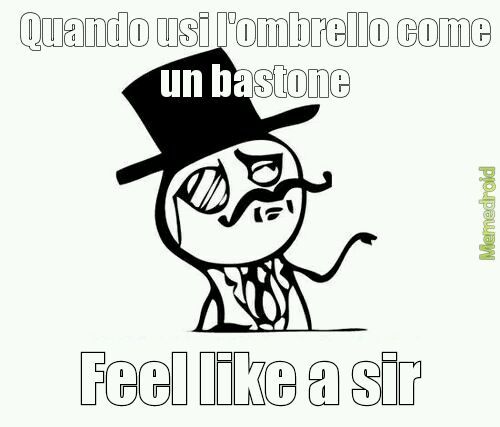The image is a black and white clipart drawing resembling a meme, featuring a character that looks like the iconic mascot of a peanut brand, often referred to as "Mr. Peanut." The character has a round face adorned with a monocle and a mustache, and he is sporting a black top hat. He has a thin, sketch-like body that only extends down to the waist, showing thin arms and what appears to be a coat and tie without sleeves. His right arm is extended out, as if offering a handshake or expecting someone to kiss his hand. At the top of the image, there is text in Spanish that says "cuando use la umbrella como un bastón," and at the bottom, it reads "feel like a sir" in English. Additionally, the word "memedroid" is visible on the right side of the image, suggesting the origin or platform of the meme.